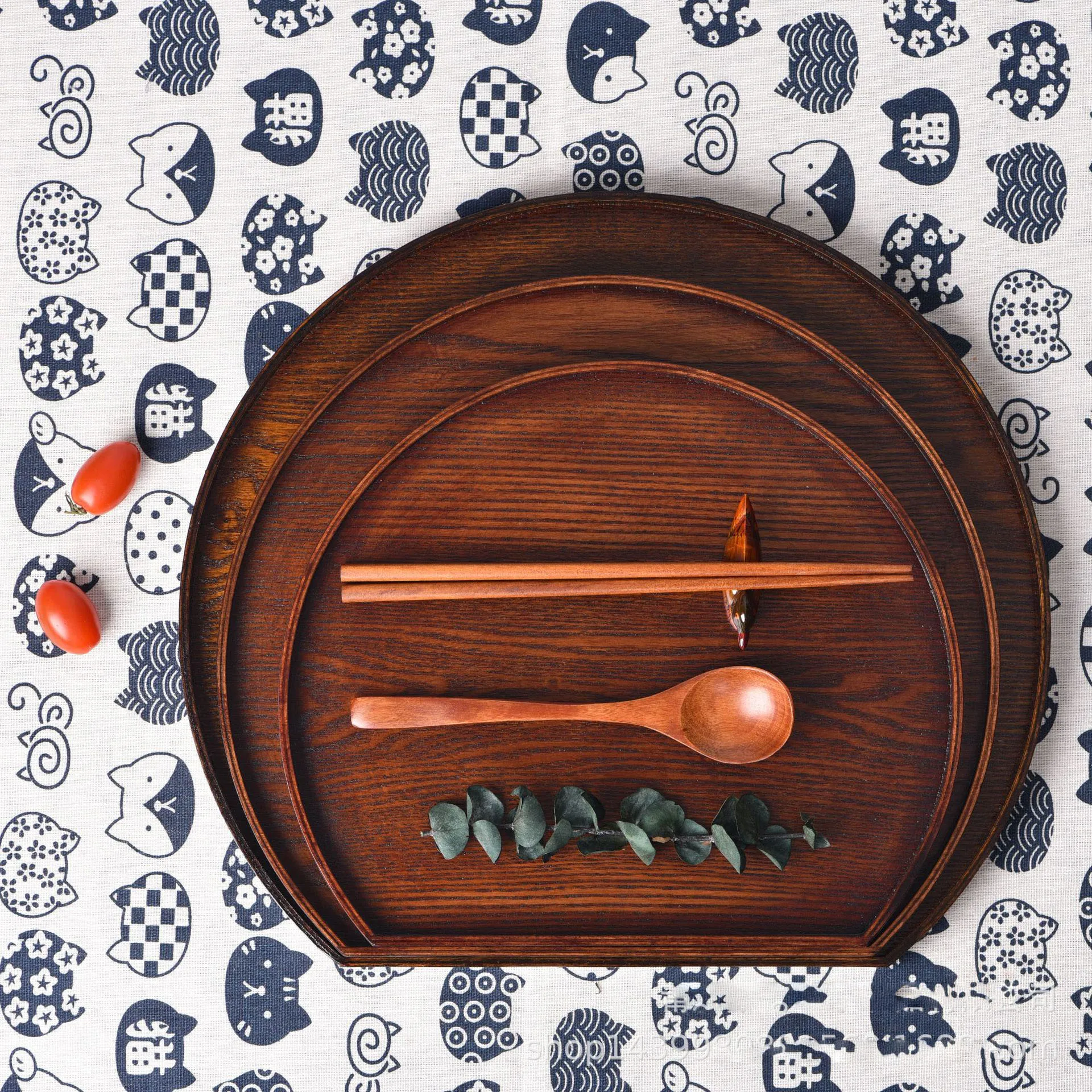This indoor photograph, shot from a top-down angle, captures a detailed arrangement on a table covered with a grey tablecloth adorned with an intricate cat pattern. The tablecloth features various cat faces, each showcasing unique designs such as flowers, scales, targets, waves, and Japanese-style text, all in playful blue hues. In the center of the image, three wooden platters of decreasing size are neatly stacked, each shaped like a circle with a flat bottom, resembling an arched design. Atop the smallest platter lies a set of brown wooden chopsticks resting on a matching wooden chopstick rest, alongside a wooden spoon. Adjacent to the spoon is a decorative twig with dried green leaves. To the left of the platters, two oval-shaped cherry tomatoes add a pop of color to the scene, completing this meticulously arranged and visually captivating setting.